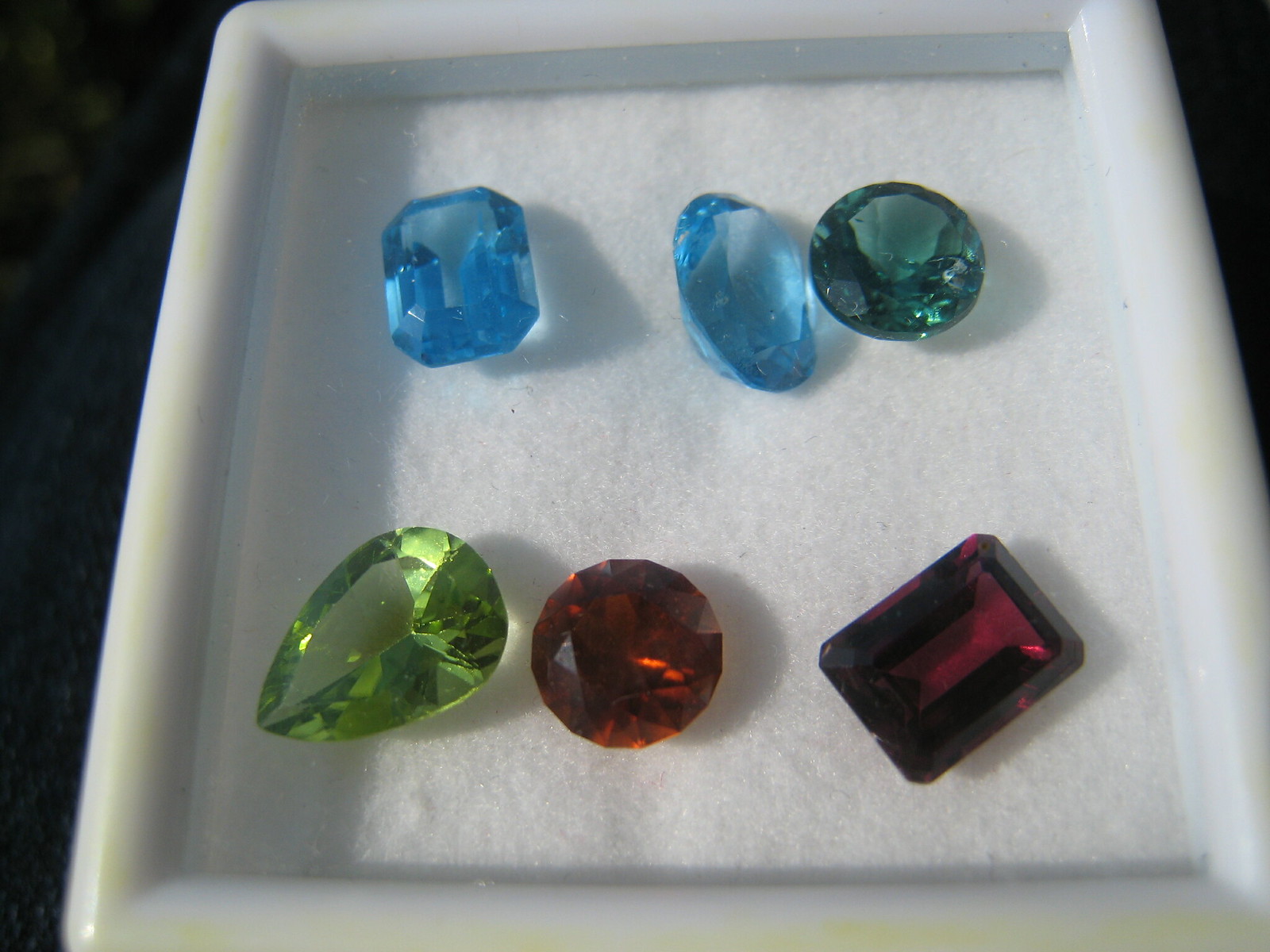This color photograph features a small, square-shaped white tray with a translucent acrylic border, placed against a black background. Within the tray is a white cotton-like base, reminiscent of snow. The tray contains six large, vividly colored gemstones arranged in two rows. On the top row, the leftmost gem is an emerald-cut aquamarine, followed by an oval-cut aquamarine, and then a circular-cut, dark green jade-like stone. The bottom row starts with a large, teardrop-shaped, light green stone, possibly a green gem, followed by a circular, dark red garnet, and finally a square-shaped, red-purple stone, with a reddish hue, towards the lower right. Each gemstone casts a slight shadow on the white surface, adding depth to their vibrant display.